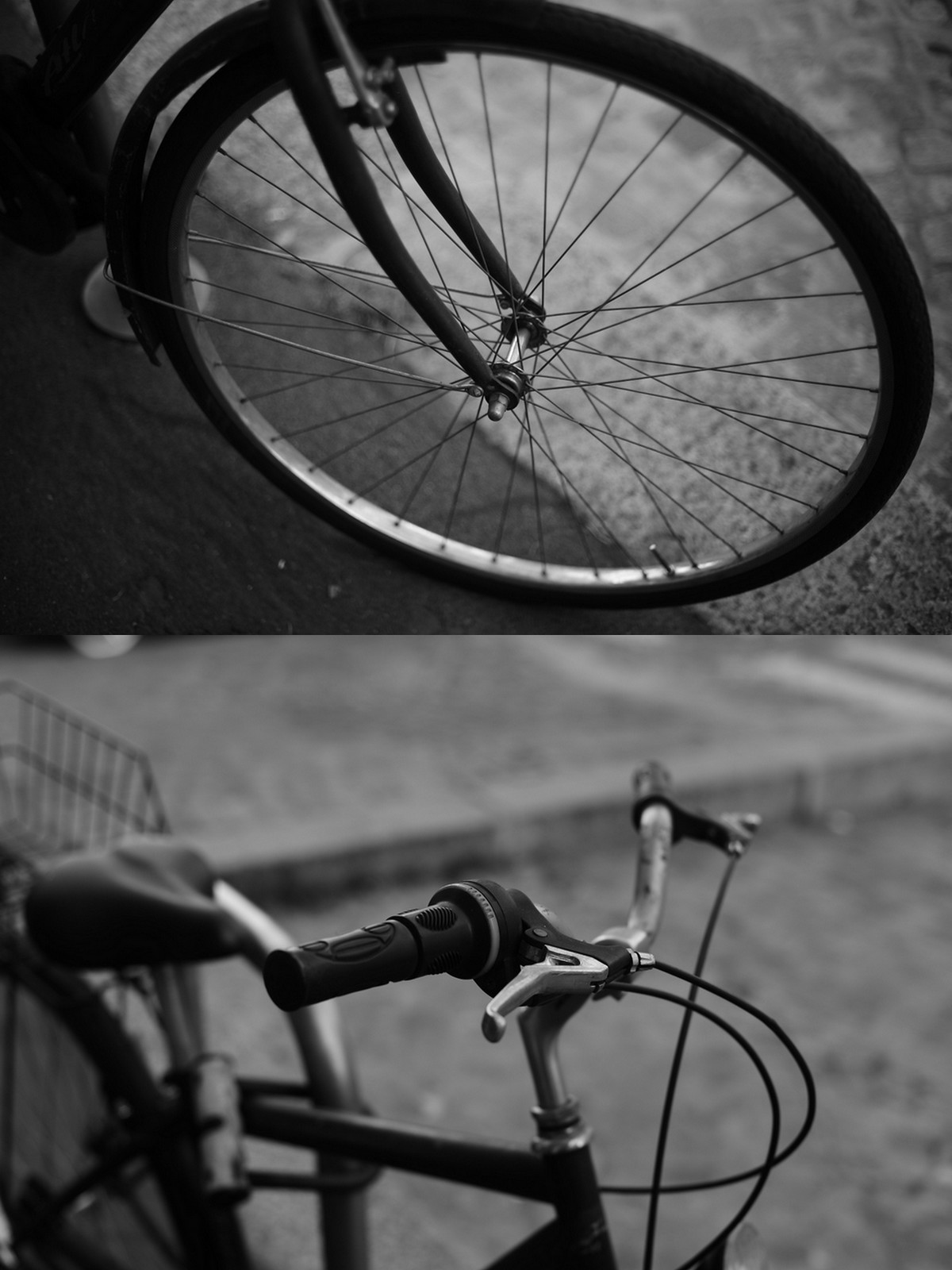This image consists of two vertically stacked black-and-white photographs, each depicting different parts of a bicycle. The upper photograph prominently features a close-up of a front bicycle wheel with distinct spokes, positioned at an angle where the top part is closer to the camera than the bottom part. This wheel rests on a paved ground that transitions from a dark gray area to a lighter gray border.

The lower photograph offers a top-down view of the bicycle's handlebar, which includes visible brake cords, and the seat. The handlebars are centrally positioned and oriented towards the bottom right corner of the image, while the seat is diagonally aligned towards the same direction, occupying the left side of the photograph. Behind the seat, a metal-frame basket or crate is mounted on the rear of the bicycle. The scene appears static, possibly indicating the bicycle is supported by a kickstand. The setting is outdoors on a street, characterized by a grayish and whitish pavement, without any textual elements or clear indications of the time of day.